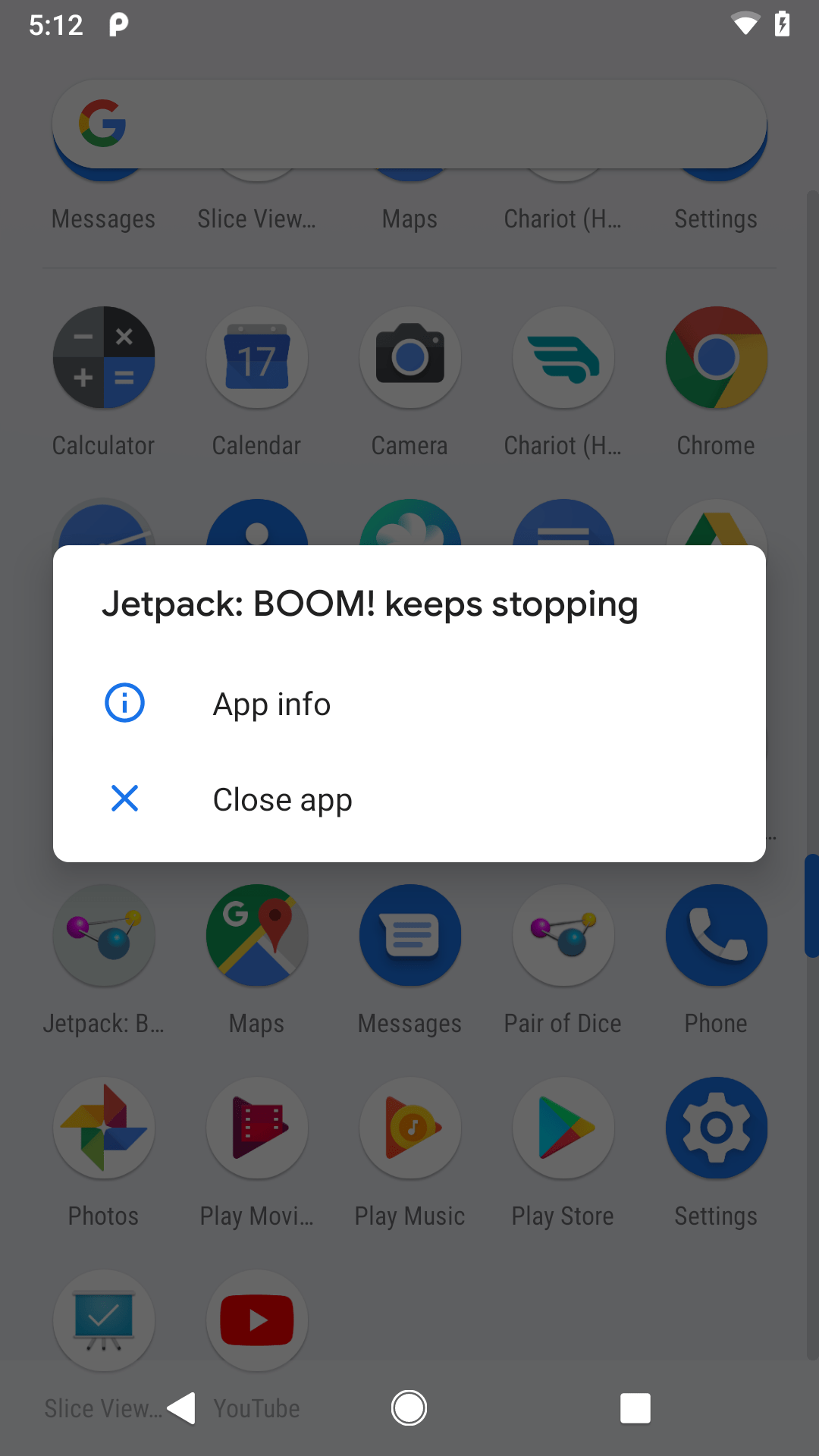In this image, we observe a mobile phone's screen displaying a pop-up message indicating an issue with an app. The notification reads, "Jetpack Boom keeps stopping," suggesting that the application has crashed. Users are given two options: "App info" and "Close app." 

At the top of the screen, the phone's status bar is visible, displaying network details, battery level, and the current time, confirming that this is indeed a mobile device.

Behind the pop-up message, the phone's home screen is partially visible, showcasing numerous app icons organised across the screen. These include: Messages, Slice View, Maps, Chariot, Settings, Calculator, Calendar, Camera, Chariot (appearing twice), and Chrome. 

Below the pop-up box, more app icons are partly obscured but identifiable. These include: Jetpack Boom, Maps, Messages, Pair of Dice, Phone, Photos, Play Movies, Play Music, Play Store, Settings, Slice View, and YouTube. The background suggests a typical smartphone interface with multiple applications readily accessible.